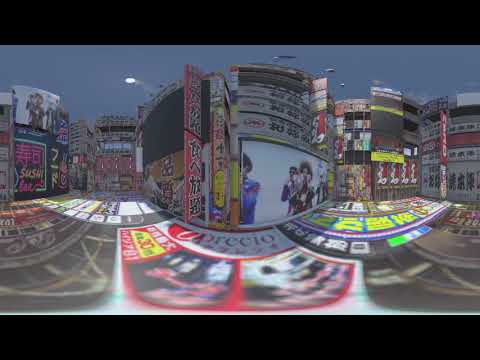The panoramic image captures a bustling street scene during dusk or evening, beneath a dark grey sky hinting at the setting or already set sun. Dominating the center of the composition are multi-storied buildings adorned with a plethora of advertisements, billboards, and vibrant signs. Central to the image is a striking billboard featuring several rock star-like figures, all sporting sunglasses and staring directly ahead. To the left of this billboard, a conspicuous large red sign with black Asian characters draws attention. The street below is unusual, with additional billboards painted directly onto its surface, creating a visually rich, albeit somewhat chaotic, urban tableau. 

The scene is characterized by a distorted or rounded appearance, possibly due to a panoramic or bubble effect from the camera, causing some nearby structures to bulge outward while distant ones appear minimized. The buildings exhibit a mix of possibly computer-generated imagery and artwork, embellished with various pictures and signs, some depicting anime characters. There are no typical street markings, and no people are visible, emphasizing the overwhelming presence of advertisements and signs, some of which are illuminated.

Among the extensive signage, one in a visible corner reads "sushi," while other texts are in Chinese or Japanese script, suggesting an East Asian urban setting. The image is framed with black headers and footers, adding to its artistic presentation. The overall scene, with its myriad of colors, texts, and illuminated elements, gives a sense of a vibrant, perhaps surreal, urban landscape rich in commercial and cultural iconography.